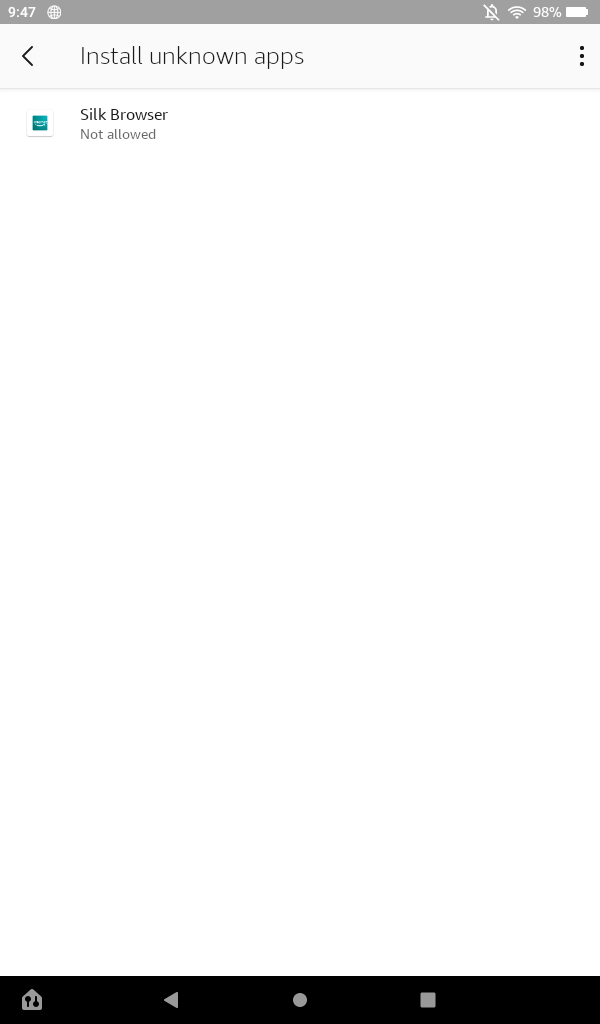A detailed screenshot of a mobile device's screen captured at 9:47 AM, indicated by the clock in the upper left-hand corner. The top section features a gray banner that includes a globe icon and a notification bell with a line through it, signaling that notifications have been silenced. The full Wi-Fi signal icon is displayed next to a battery symbol showing 98% battery life. A left-facing back arrow is present in the black background of the top section. Centered on this black header, the text "Install unknown apps" is prominently displayed. To the right of this text, three vertical black dots are visible, typically indicating additional options. Below this header, a gray divider separates the main content. The primary content area shows the text "Silk browser not allowed" accompanied by a small square blue box icon. The banner at the bottom, featuring a black background, includes icons linking to the home screen and for navigating back.